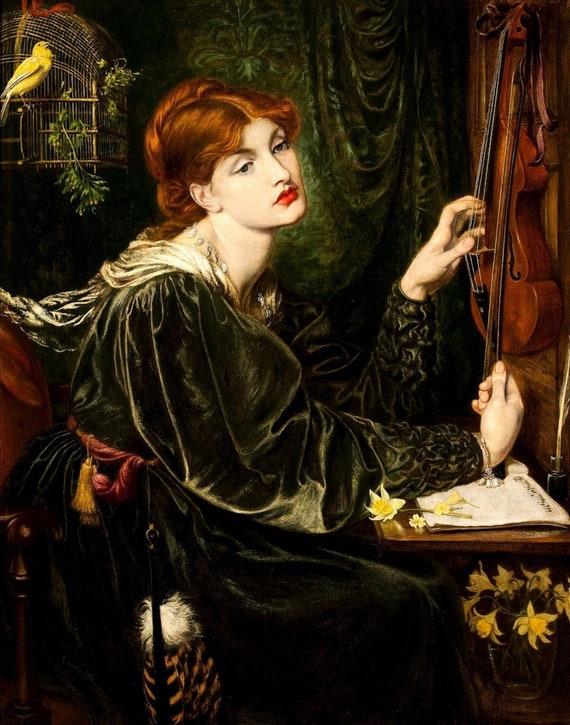In this Renaissance-inspired painting, a fair-skinned woman with striking red hair and vivid blue eyes sits serenely, gazing wistfully towards the bottom right of the image. Her red hair is elegantly parted in the center and pulled back, accentuating her melancholic expression highlighted by her bold red lipstick and pronounced bottom lip. She is dressed in a sumptuous olive green, velvety gown tied at the waist with a red cord, and she dons a necklace adorned with seashell-like accents.

Seated at a table, she delicately plucks the strings of a violin hung on the wall before her with her left hand, while her right hand gently holds the bow. A glass vase filled with vibrant yellow flowers rests on the floor by her knees, and more yellow flowers adorn the table supporting her right arm. Above her head, in the left section of the image, a yellow bird perches inside its cage, adding a touch of whimsy to the dark, black background that frames the scene. To the back of her, a green curtain subtly hangs, softly contrasting with the other elements in the painting.